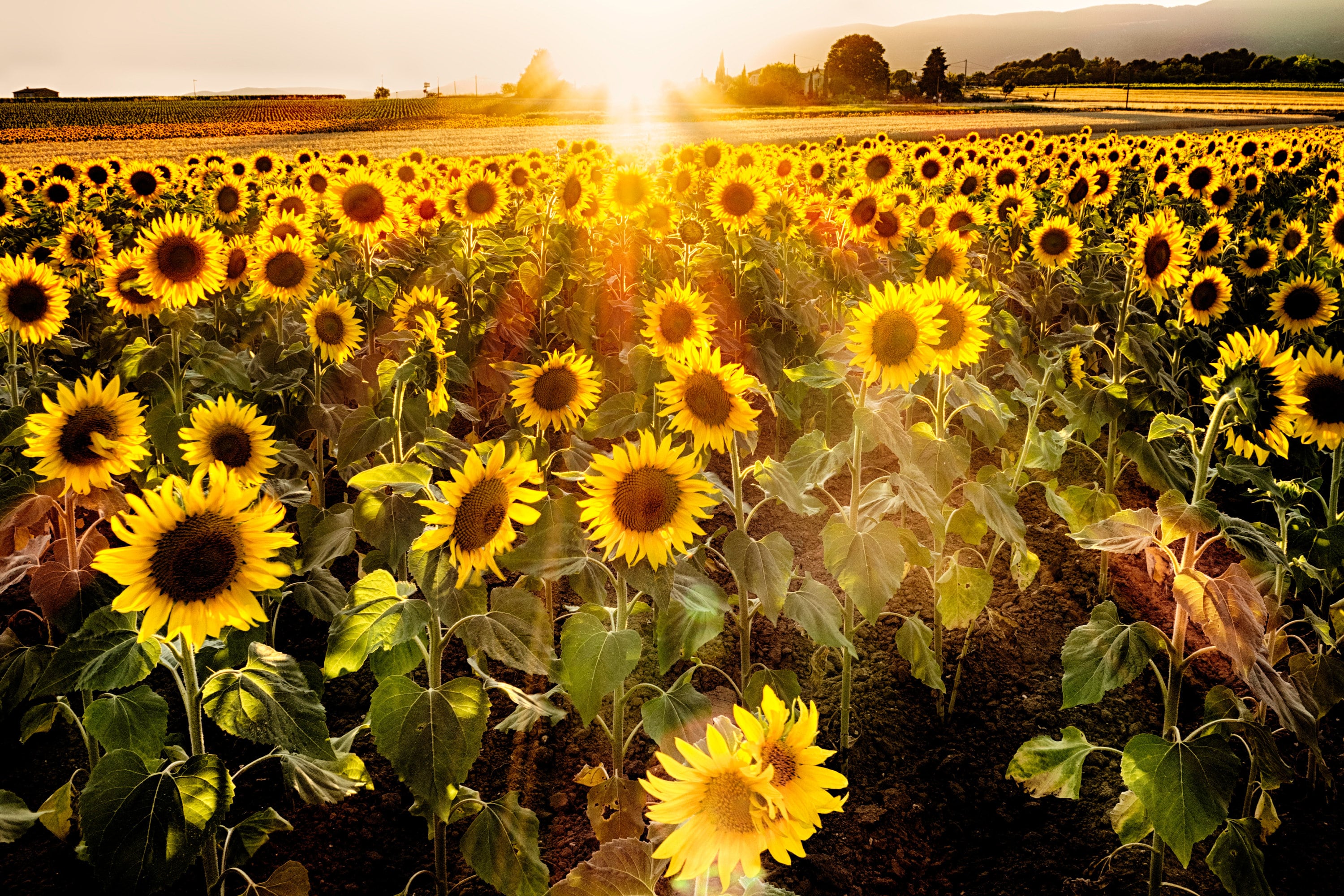This photograph captures the serene beauty of a vast sunflower field, the vibrant yellow petals and brown seeds standing out against the green stems and leaves. Dominating the foreground, hundreds of tall sunflowers, reaching up to mid-waist height, seem to face towards us, almost basking in the golden light of the setting sun. The sun itself, positioned in the top center of the image, stretches its warm rays across the scene, casting a magical glow over the entire field.

Just behind the sunflower expanse lies an empty, light yellow field, devoid of any growth, creating a stark contrast and a visual transition to the subsequent cornfield further back. On the right side, a cluster of trees lines a dirt road, interspersed with power lines. These trees extend towards a distant hill or mountain adorned with more green trees, adding depth to the landscape.

A house is faintly visible on the very top left, subtly blending into the vastness of nature. The sky above is a clear expanse, free of clouds, enhancing the pure and unblemished ambiance of this rural panorama.